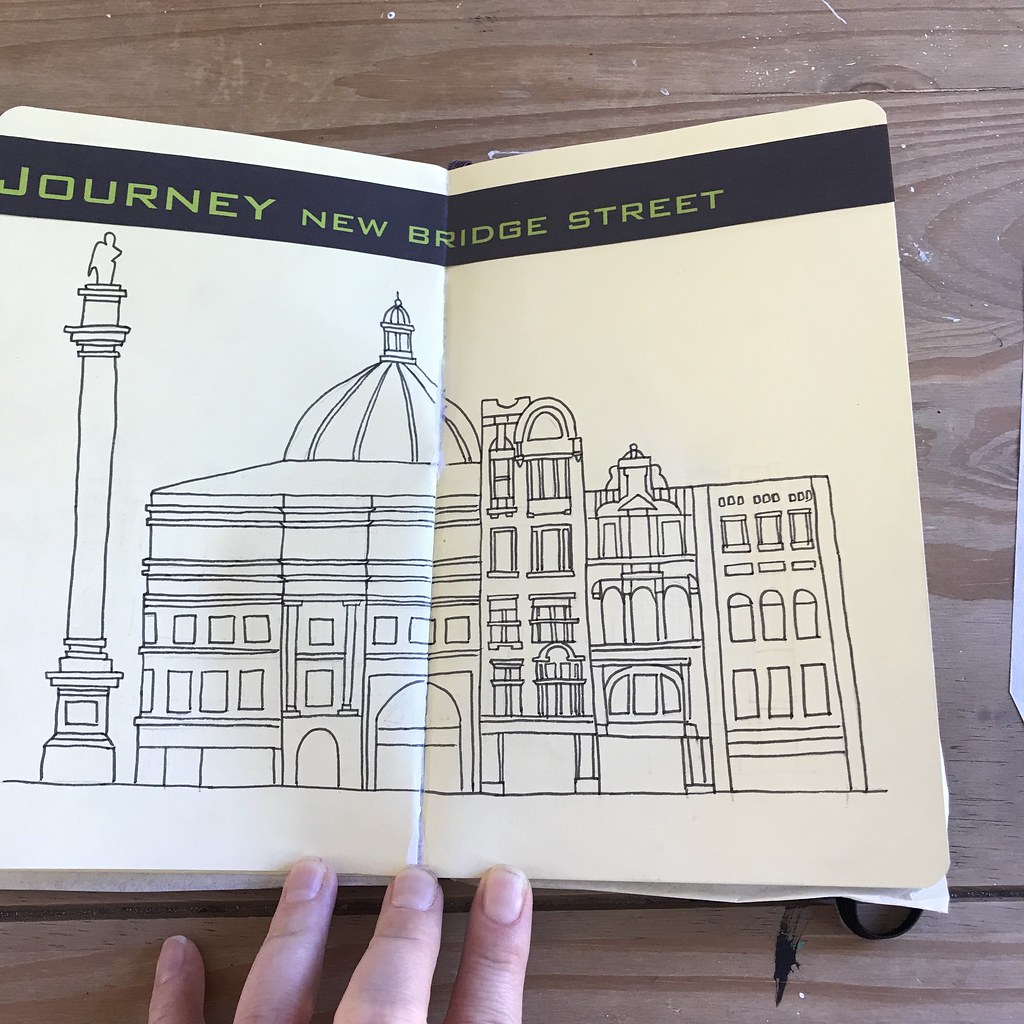In this image, there is an open book resting on a wooden table. The book is positioned so that a left hand is visible in the bottom left corner of the frame, suggesting someone is holding or steadying it. The page on display features a hand-drawn illustration rendered in black ink on white paper. At the top of the page, inside a blue box with green text, the title reads "Journey New Bridge Street."

The drawing showcases a streetscape with several structures. On the left side, there is a monument or pole with a distinct design at its summit. Adjacent to this, there appears to be a church, characterized by its architectural features. Further to the right, there are additional buildings that look like residential houses. The style of the drawing is simple and straightforward, indicating a modest level of artistic skill.